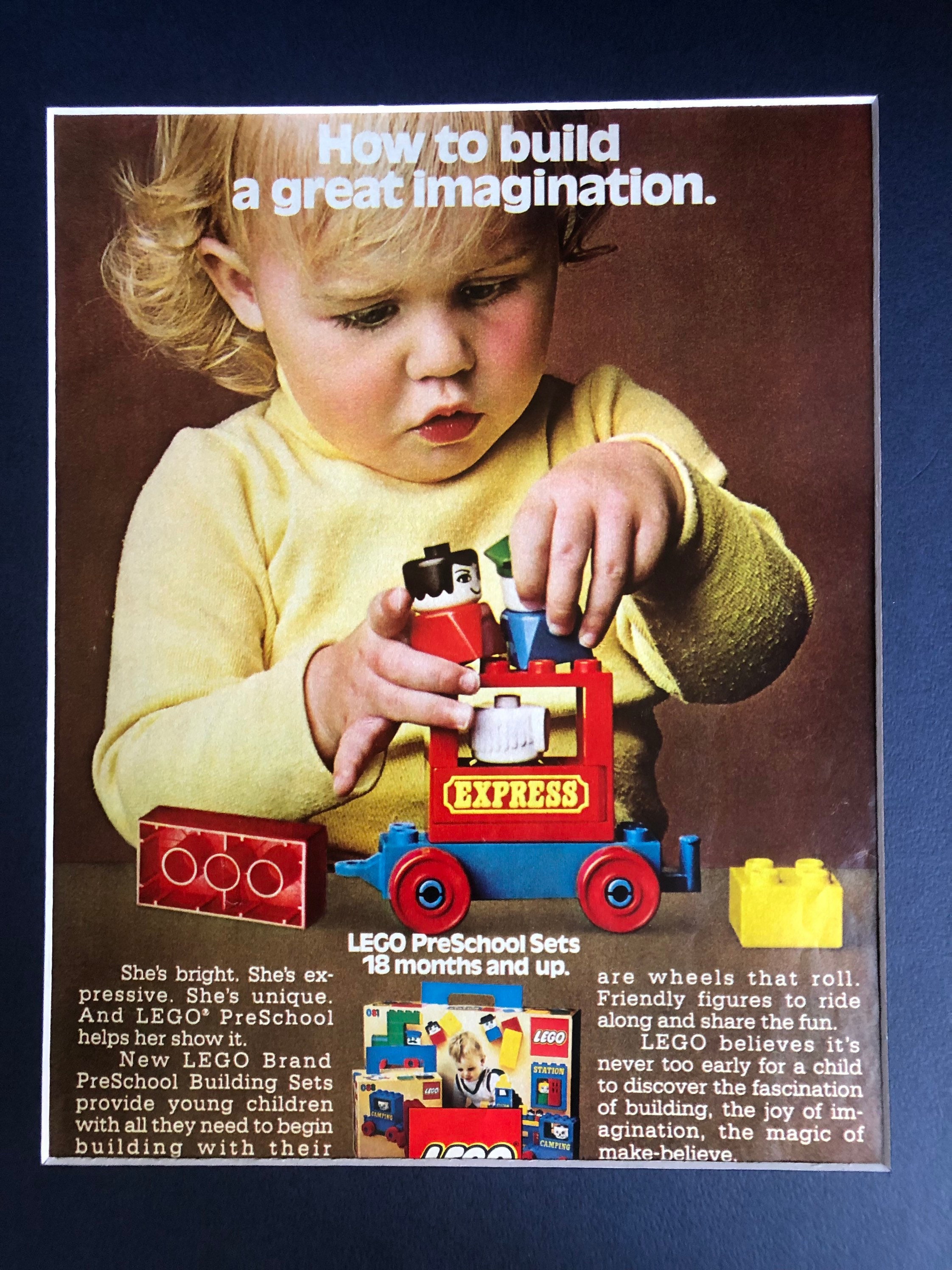The colorful advertisement showcases a bright and cheerful scene of a young girl with light skin and blonde hair, immersed in play with a Lego preschool set. The girl, dressed in a yellow tank top, is animatedly assembling a vibrant toy train, which prominently features red and blue colors with the word "Express" emblazoned in yellow letters on its side. A friendly toy figure is perched atop the train, adding to the playful atmosphere. Surrounding the train are various Lego pieces, including noticeable red and yellow blocks, bringing the setup to life.

Above the scene, in striking white letters, the caption reads, "How to build a great imagination." Below the girl, the center of the image displays the logo with two columns of text bordering it, stating, "She's bright, she's expressive, she's unique and Lego preschool helps her show it," accompanied by a smaller caption detailing, "New Lego brand preschool building sets provide young children with all they need to begin building their own wheels that roll, friendly figures to ride along and share fun with." The clarity of the image is enhanced by natural lighting, contributing to the overall bright and inviting setting, appealing to parents and children alike.